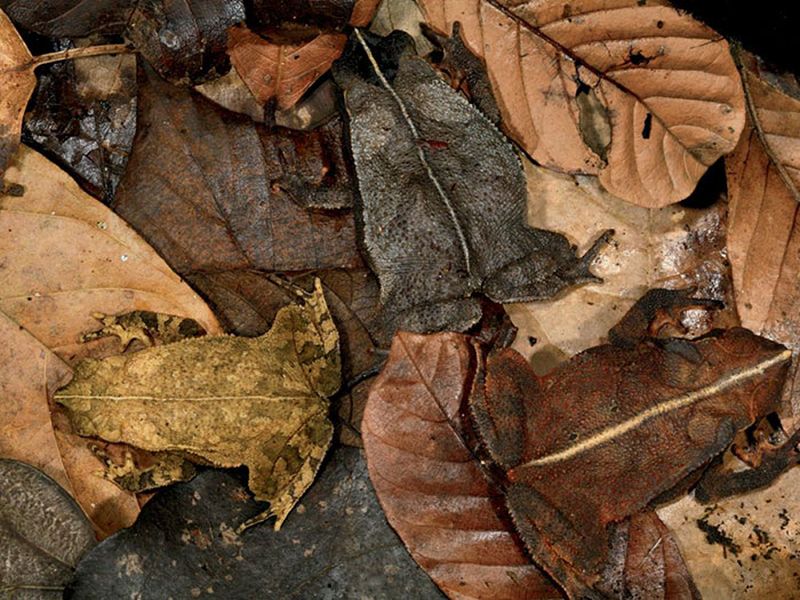This close-up photograph vividly captures a trio of masterfully camouflaged toads on a forest floor strewn with dried, crumpling leaves in varying shades of grey and brown. Blending seamlessly into their natural surroundings, which are slightly moist and appear to be taken outdoors in daylight, these toads remarkably resemble the fallen leaves they rest upon. 

To the top center, a grey toad with subtle black speckles and a light whitish-yellow spine subtly hides beneath similar-colored foliage, making it nearly indistinguishable from its surroundings. On the left, a yellow toad with hints of green blends with adjacent yellowing leaves, its leaf-like shape and patterns camouflaging it effortlessly. The right side features a maroon toad whose color and texture mimic the brown, decayed leaves beside it, further enhancing its disguise. 

Each toad lays amidst the grey and brown leaf litter, their body's leaf-like shape and detailed patterns reinforcing their camouflage and making it a challenge to differentiate these wildlife creatures from the forest debris they inhabit.